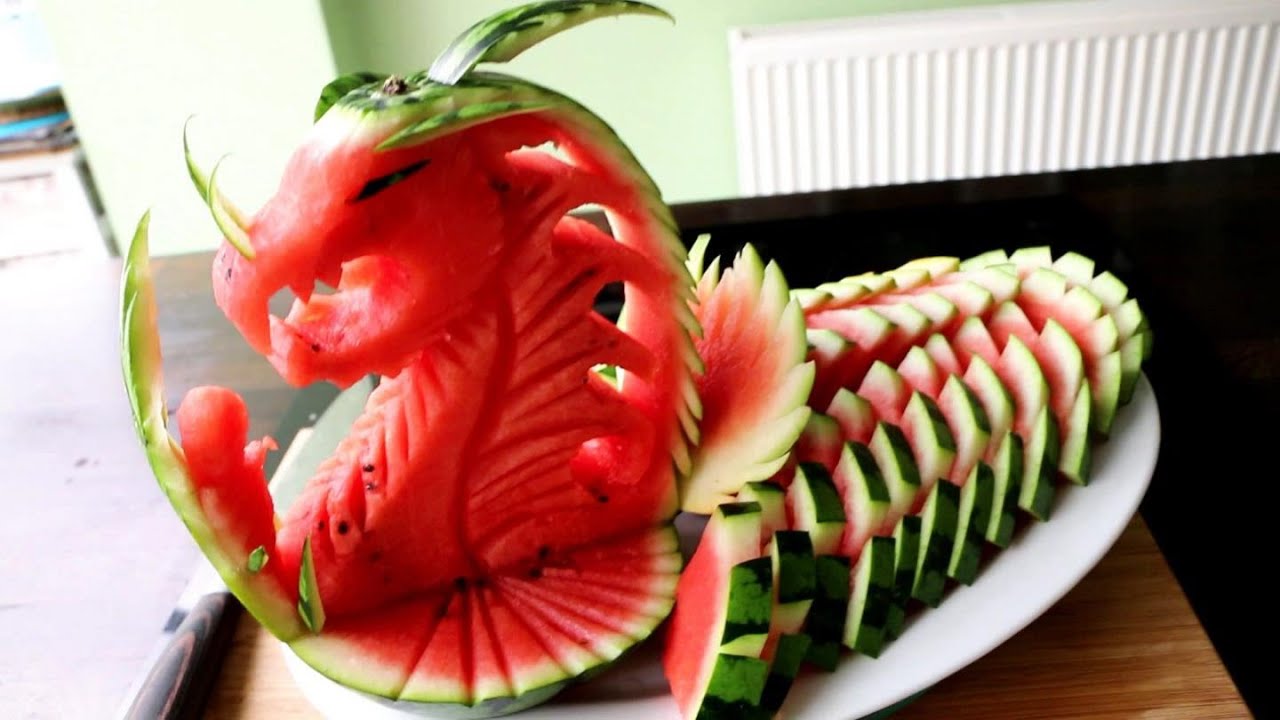The photograph depicts a meticulously crafted fruit sculpture against a light green wall, wherein a watermelon has been artistically carved to resemble a dragon. Positioned on a white oval platter atop a brown table, the dragon's head is oriented to the left, showcasing the vivid red flesh of the watermelon. The head features intricate details, including two curled green peels forming the dragon’s nostrils, an open mouth with sharply defined teeth, and a black slash mark representing an eye. The dragon’s body extends to the right in vertical sections, maintaining the overall shape of the original watermelon, with green and black peel segments forming a spiked effect along the top and sides. A green tuft accents the top of the dragon's head, adding to the lifelike appearance. The use of watermelon seeds to create the eyes further enhances the detailed craftsmanship of this elegant and elaborate fruit sculpture.